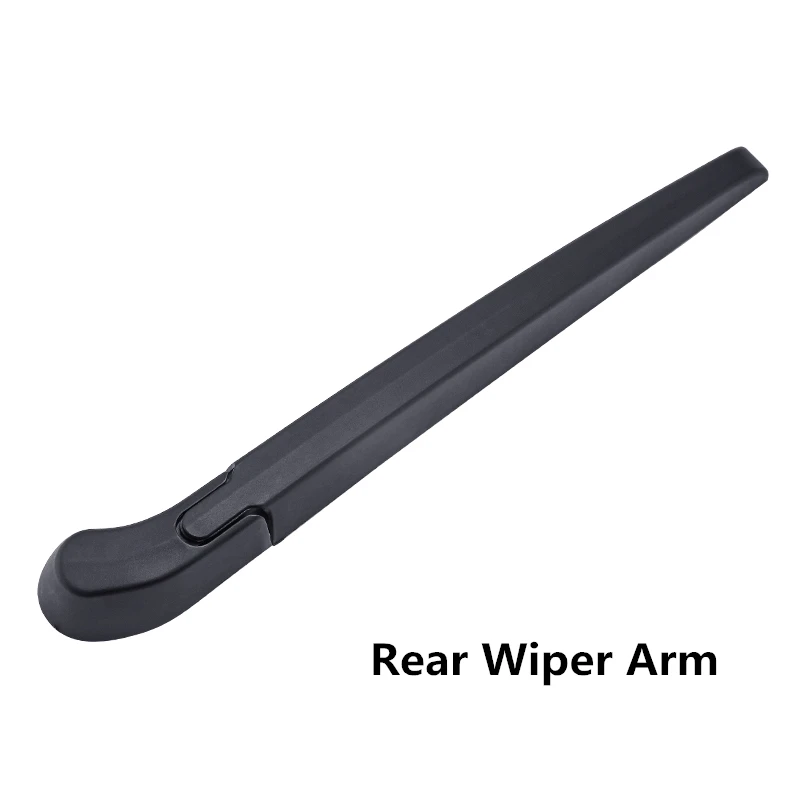The image depicts a rear wiper arm on an all-white background with the text "REAR WIPER ARM" written in black at the bottom, with each word capitalized. The wiper arm, made of plastic and colored in a very dark gray or black, spans diagonally from the rounded bottom left to the narrower top right. The arm features a subtle ridge along its center, running lengthwise from the wide, slightly curved base to the tapered top. A noticeable U-shaped connection area with a small oval cutout is located towards the bottom left, highlighting where two pieces are joined together. The overall shape of the wiper arm is three-dimensional, curving gently and adding depth to its form.